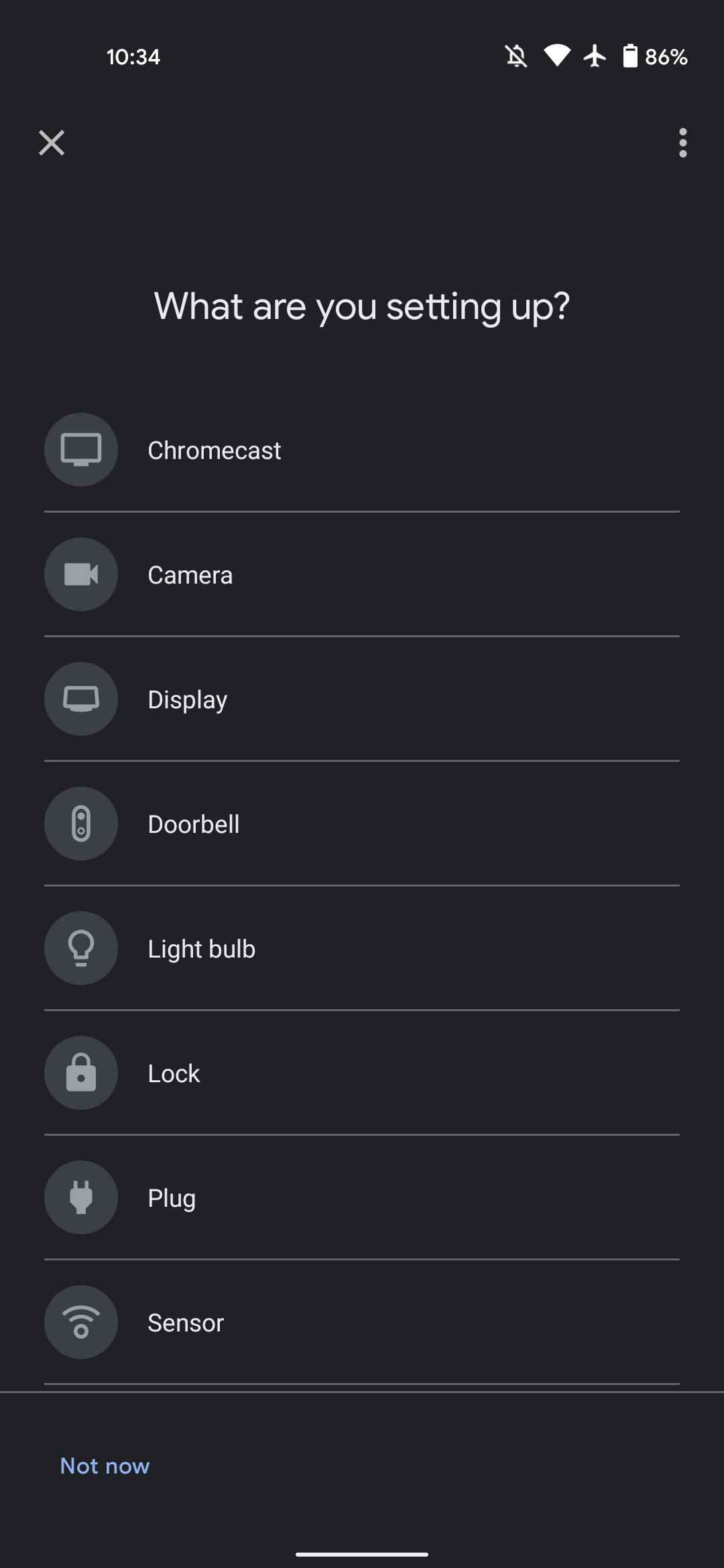A cell phone screen displaying a setup menu with a black background and predominantly white text. 

In the upper left corner, "10:34" is shown. To the right, icons indicate that the notification bell is off, Wi-Fi is on, and airplane mode is activated, along with an 86% battery life indicator.

Below this, a horizontal line separates the top informational section from the central menu area. On the left side of the line, there's an 'X' icon; on the right, three vertically aligned dots. In the middle, text reads, "What are you setting up?" 

Beneath the question is a list of device categories, each accompanied by an icon:
1. Chromecast - represented by a television screen icon.
2. Camera - depicted as a video camera.
3. Display - symbolized by a computer monitor.
4. Doorbell - shown as an oval with two vertical dots.
5. Light bulb - illustrated as a traditional light bulb.
6. Lock - represented by a padlock.
7. Plug - illustrated by an electric plug.
8. Sensor - shown as a circle with V-shaped lines radiating upwards.

Each category and icon are left-justified, with a gray line separating each item. At the bottom left, in blue text, is the option "Not now." In the bottom center of the screen is a white bar. 

The visual elements are limited to black, white, gray, and blue, providing a clean and simple interface.